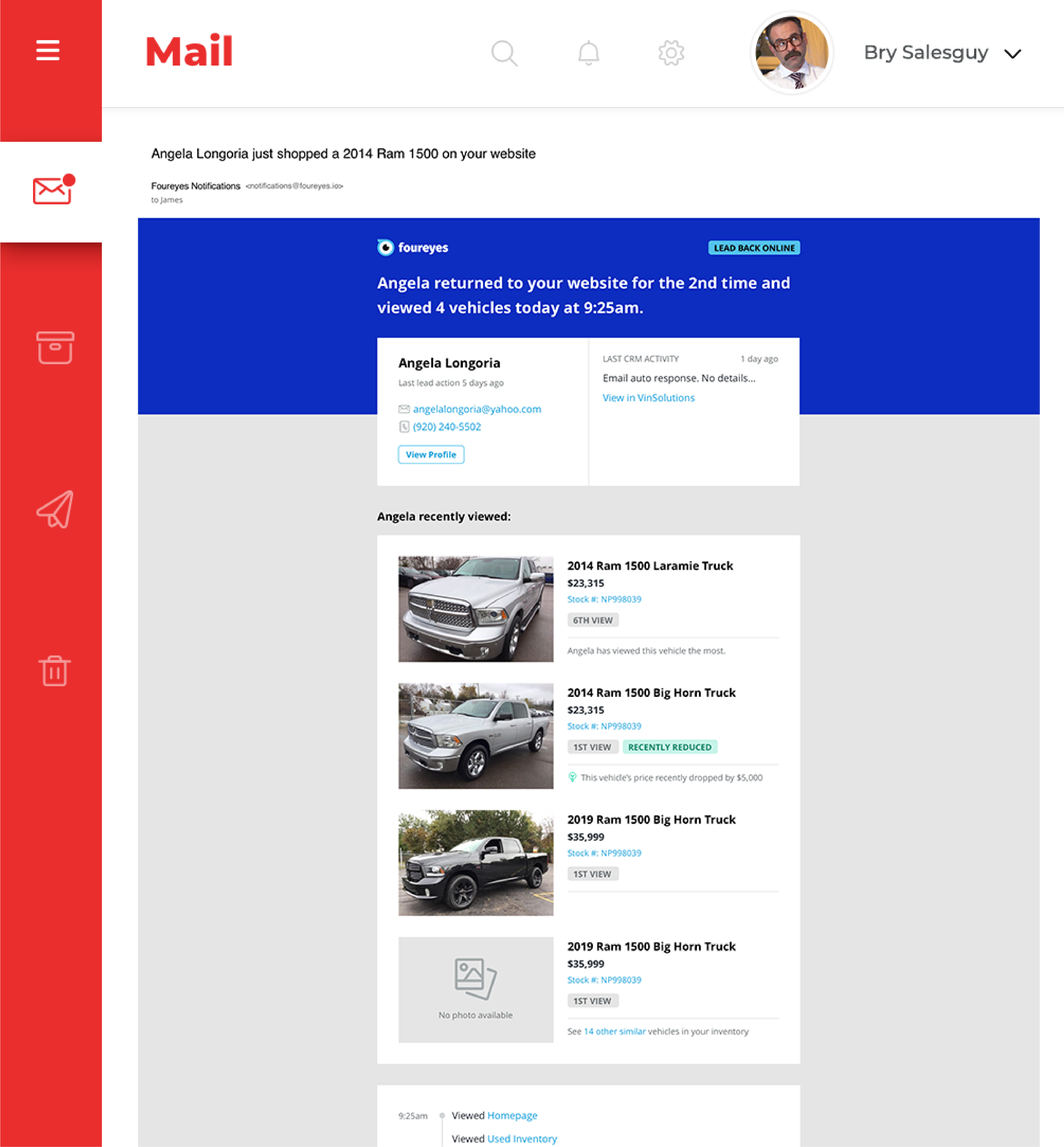In the image, we see a screenshot that appears to be from a sales or customer interaction interface. In the upper right corner, there is gray text that reads "Bry Sales Guy," accompanied by an image of a man with dark glasses, a mustache, and dark hair. He is wearing a white collared shirt and a tie. In the upper left corner, a red rectangle contains three short horizontal lines, likely representing a menu icon. 

Next to this rectangle, on a white banner, the word "Male" is prominently displayed in bold red text. Beneath the banner, in smaller black text, is the name "Angela Lingoria," with an accompanying note that she recently shopped for a 2014 Ram 1500 on the website.

A large blue banner below this section shows the phrase "Four Eyes" in white text, indicating that Angela returned to the website for the second time and viewed four vehicles today at 9:25 a.m. Additionally, in the upper right, there is a small light blue box containing black text that reads "Lead Back Online," possibly indicating a status update for the sales lead.